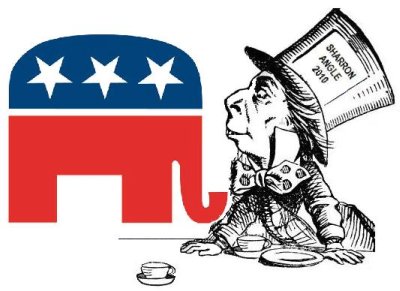The image appears to be a political cartoon set against a white background. On the left side, there's the Republican elephant emblem, featuring a blue top adorned with three white stars and a red lower half, complete with a trunk and legs. On the right side, there is a black and white sketch of a man resembling the Mad Hatter from Alice in Wonderland. The character is depicted wearing a tall top hat labeled "Sharron Angle, 2010" and a large, spotted bow tie. Positioned in front of him is a table set with a couple of teacups and a plate. The Mad Hatter-like figure is captured in profile, facing and seemingly focused on the Republican elephant emblem.